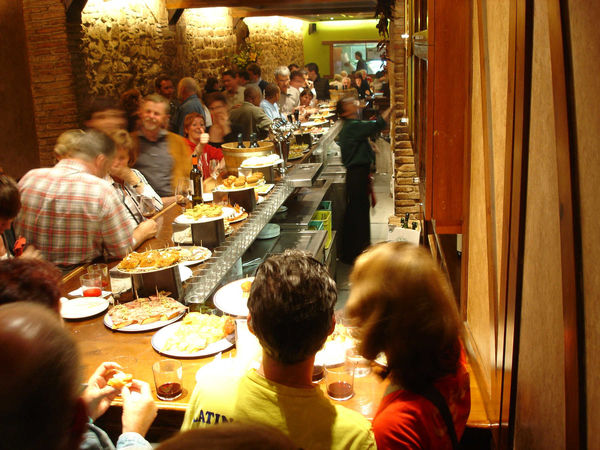The photograph captures a bustling scene at a restaurant bar, viewed from a landscape orientation. The long wooden bar stretches from the bottom left, slightly upwards to the right, dominated by an array of glasses filled with drinks and plates of various hors d'oeuvres on risers. Positioned in the foreground, toward the bottom middle of the image, is a person with short dark hair in a yellow t-shirt seated facing away from the camera. To their right is another individual in a red shirt with shoulder-length, reddish-brown hair. A third person is partially visible behind them, with just the top of their head and hands reaching forward, holding something.

The bar area is lively, with around 20 patrons both standing and sitting, absorbed in conversation and dining. The middle of the bar, marked by a basket containing bottles, indicates a midpoint in the image. To the right, where the bar continues into the background, the scene remains cluttered with drinks and food, reinforcing the vibrant activity.

Behind the bar, metal surfaces and small crates are visible, adding a functional backdrop to the scene. A somewhat blurry figure in a green shirt and black pants works behind the counter, looking to the right, possibly engaged in preparation. To the left side of the image, the presence of people and some overhead lighting makes this area a bit fuzzy, contrasting with the clearer right side which features a distinct brown wall.

Ceiling beams and a wall made of rock and brick frame the setting, contributing to the rustic and cozy atmosphere. Despite the overall blurriness of the photo, particularly in the faces of the people, the image effectively captures the dynamic and immersive environment of a restaurant bar.